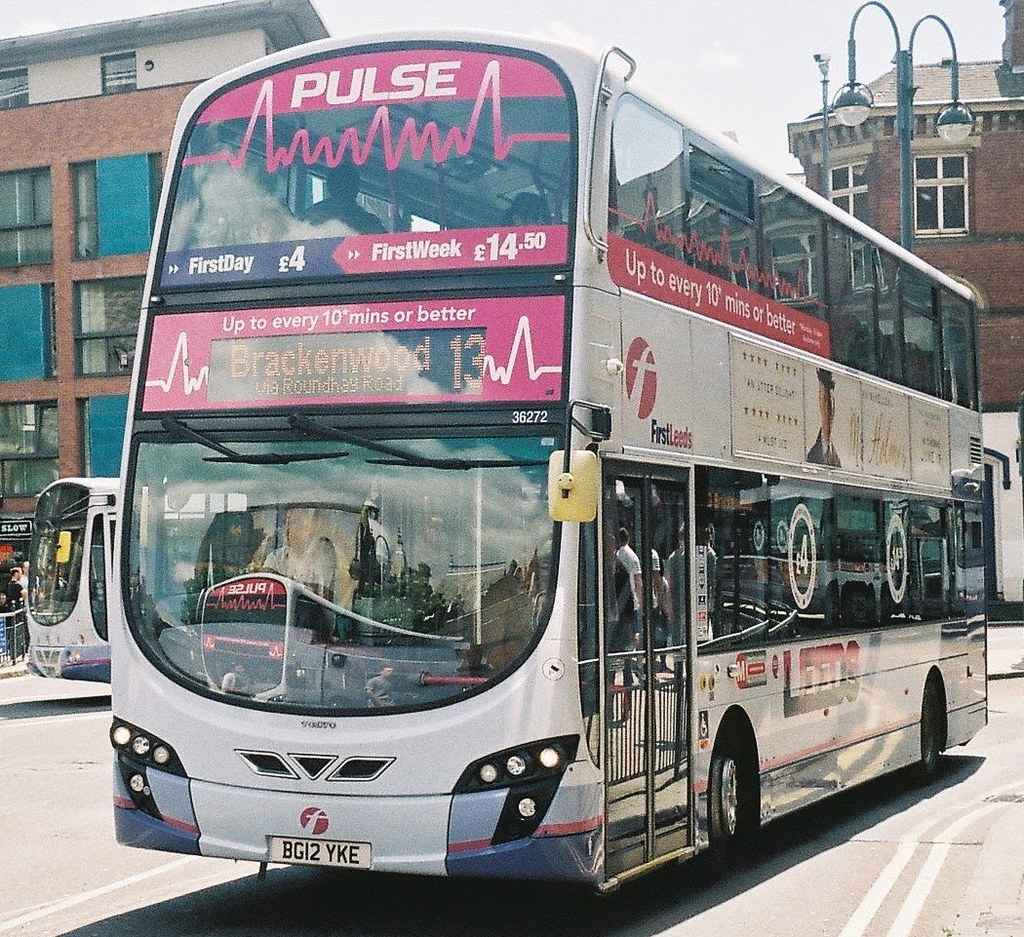This detailed outdoor photograph captures a bustling city street lined with buildings. Dominating the scene is a white double-decker bus, prominently displaying the route number 13 to Brackenwood via Round Hog Road. The bus, with its right-hand-side steering wheel, features a striking pink horizontal strip at the top front with the word "PULSE" emblazoned on it, accompanied by additional advertisements detailing fare information: "First day £4, first week £14.50, up to every 10 minutes or better." The bus's license plate reads BG12YKE. Just ahead, another bus can be seen at a slightly different angle, adding to the dynamic urban atmosphere.